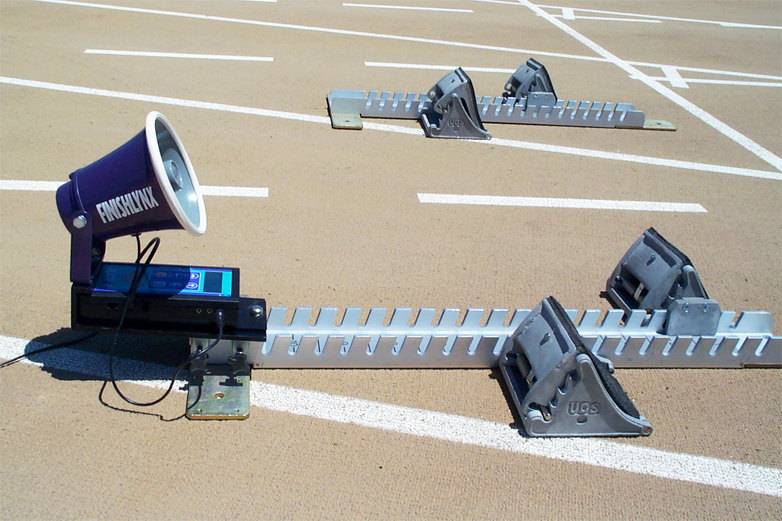The photograph displays an outdoor scene, likely on a test ground or track field, featuring intricate mechanical equipment laid out on a clean, beige-ish surface with white painted lines. Central to the image is an apparatus labeled "FINISH LYNX" in white text on a dark blue or purple megaphone-like device, electronically attached to a box. Adjacent to this are lengthy metallic tracks embedded with teeth and flanked by triangular mechanical blocks, possibly jack stands. These structures extend across the pavement, which appears to be illuminated by sunlight, highlighting their silver and metal components. In the background, a simplified version of the apparatus without the electronic box can be seen, consisting solely of a metal rod with similar teeth and triangular calibrations. The precise purpose of these mechanisms is unclear, but the detailed arrangement on the pavement suggests they're part of a sophisticated setup, possibly related to track and field measurements or timing systems.